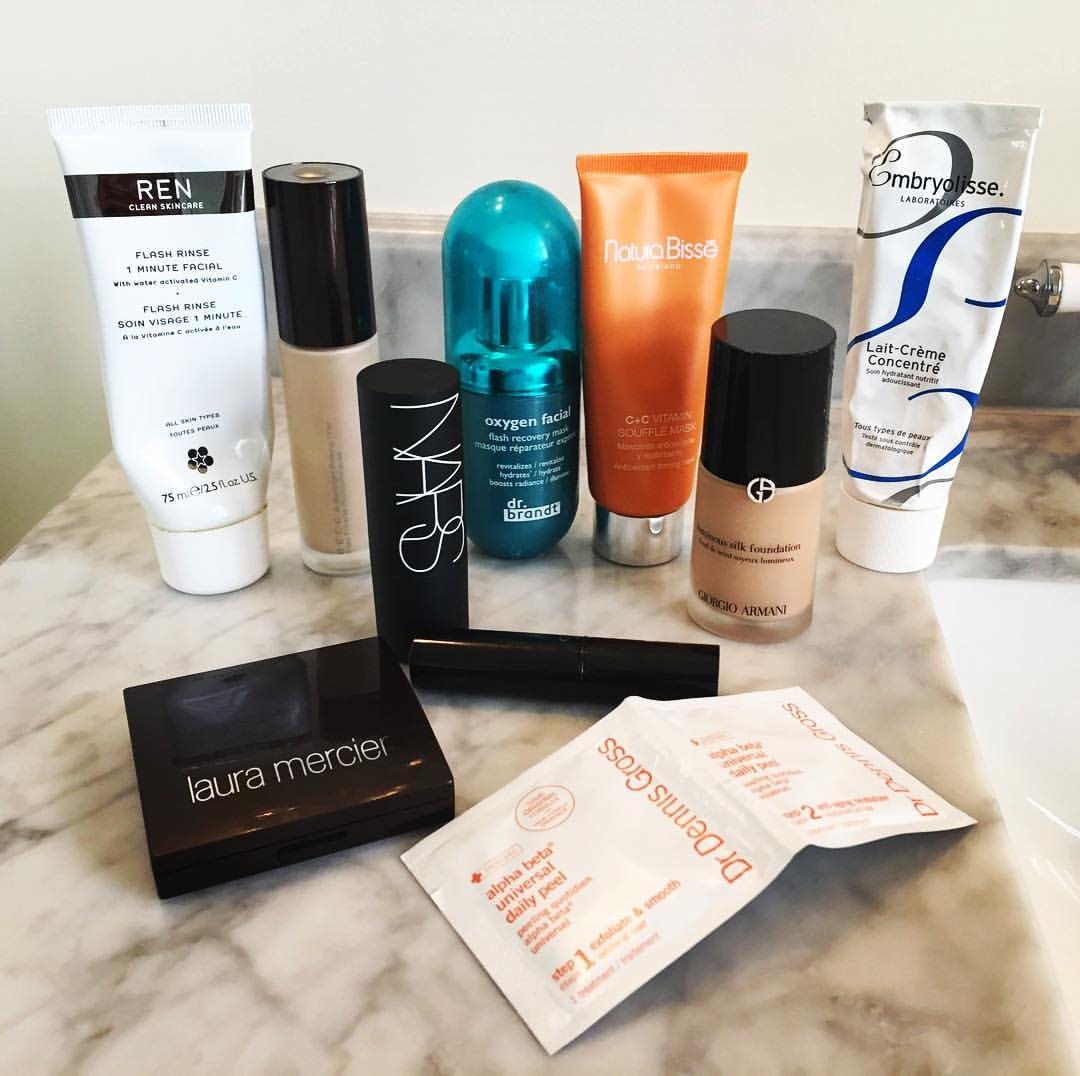A meticulously arranged collection of personal care items is displayed on a pristine marble countertop in a spacious bathroom. Dominating the foreground is a gleaming white tube labeled "R.E.N. Flash Rinse Woman Official." Nearby, a small tube that resembles a nail polish container is visible. Standing upright is a sleek black tube of NARS lipstick. Beside it lies another lipstick tube. 

A rectangular, black box with "Laura Mercier" elegantly inscribed on it takes a central position, adding a sophisticated touch. In front of this, a compact double packet labeled "Alpha Beta Universal Daily Peel" by Dr. Dennis Gross stands out with its white and orange design. An orange tube marked "Paula's Choice" is also prominently displayed, resting on its cap.

Adding a splash of color, a green tube labeled "Oxygen Facial" can be seen. To the far right, almost blending into the background, is a tube of "Embryolisse," completing the diverse array of beauty and skincare products. Just at the edge of the countertop, a white inset sink is partially visible, hinting at the bathroom setting. This carefully curated assortment of lotions and cosmetics reflects a thoughtful beauty regimen.